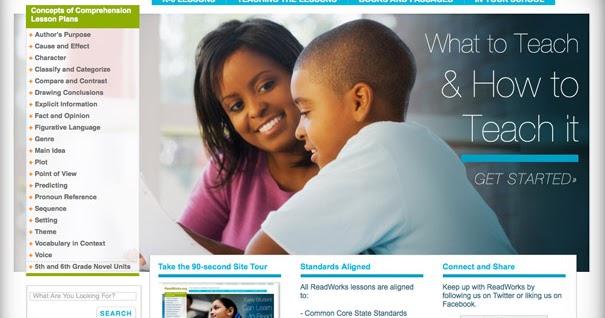The image is a partial screenshot from a website and has a horizontally rectangular frame. It is dominated by a large, horizontally rectangular image with a right indent. The image shows a smiling woman facing the viewer, while a child in the forefront looks down towards the left. The woman’s gaze is directed at the child, implying an interaction or moment of connection. Overlaying the image on the right side is text that reads, "What to teach and how to teach it. Get started."

On the left side of the frame, there is a vertical rectangle with a white background that lists various selections related to comprehension lesson plans. The list includes detailed topical themes, such as author's purpose, cause and effect, character, classify and categorize, compare and contrast, drawing conclusions, explicit information, fact and opinion, figurative language, genre, main idea, plot, point of view, predicting, pronoun reference, sequence, setting, theme, vocabulary and context, voice, and 5th and 6th grade novel units.